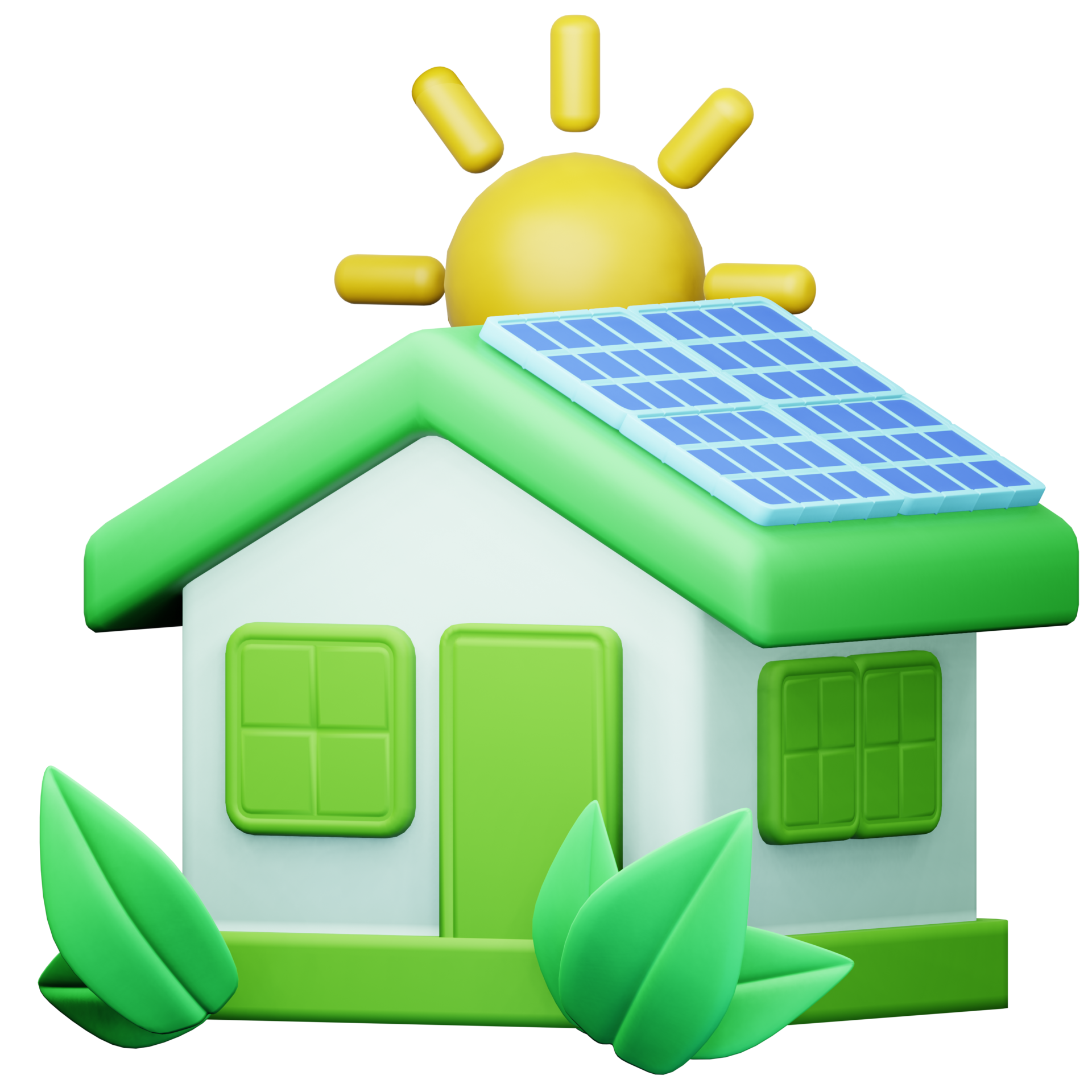This image depicts a 3D-generated design of a minimalistic toy house. The house, painted white, features a vibrant green roof and green-colored doors and windows. Two windows, comprised of smaller green squares, are positioned with one at the front and another on the side. The house stands on a green base, next to which large, translucent green leaves—five in total—are arranged, with three leaves on the right side and two on the left. Blue solar panels, represented by blue grids within larger blue squares, adorn the triangular roof. A decorative yellow sun, styled as a spherical plastic ball with protruding rays, is visible in the background. The entire composition is set against a white backdrop, emphasizing the polished, smooth texture and simplistic, computer-generated aesthetic of the toy-like object.